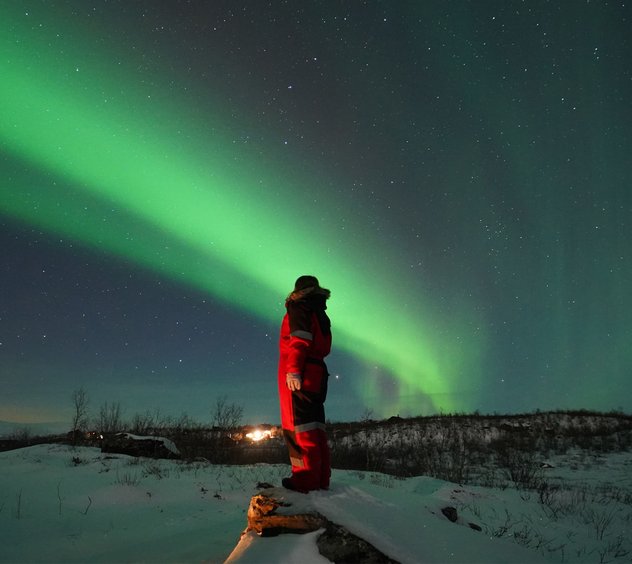In this captivating image, a person bundled up in a red snowmobile suit and a fur-lined parka hat stands on a snowy, slightly rocky overlook, gazing at the mesmerizing Aurora Borealis. The scene takes place in a frigid, northern region, possibly the Antarctic, under a dark blue night sky peppered with brilliant stars. The individual, their back to the camera and hands hanging at their sides, is set against a backdrop of a fluorescent green aurora streaking diagonally from the bottom right to the upper left of the photograph. Near the ground, the aurora features a green ring that fades as it ascends. In the immediate surroundings, there is a small campfire with flickering flames, encircled by patches of dark vegetation scattered across the snow-covered landscape.